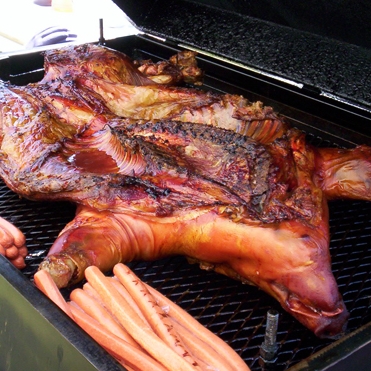The image depicts a detailed close-up of a rectangular barbecue grill, with a half pig splayed out, belly up, and charred to a crispy finish. The pig, still with its face and snout visible in the bottom right corner, is cooked to a rich mix of pink, brown, and yellow hues, with areas of deep grey or black charring. Surrounding the pig are numerous thin, pink hot dog sausages, some placed in a neat pile at the center while others are scattered along the sides. The grill grates below are black, and the barbecue itself has a dark green outer side, with its lid partially visible and matching the grill's dark color. The scene is brightly lit, suggesting it's daytime, with light streaks visible in the top left corner of the image.